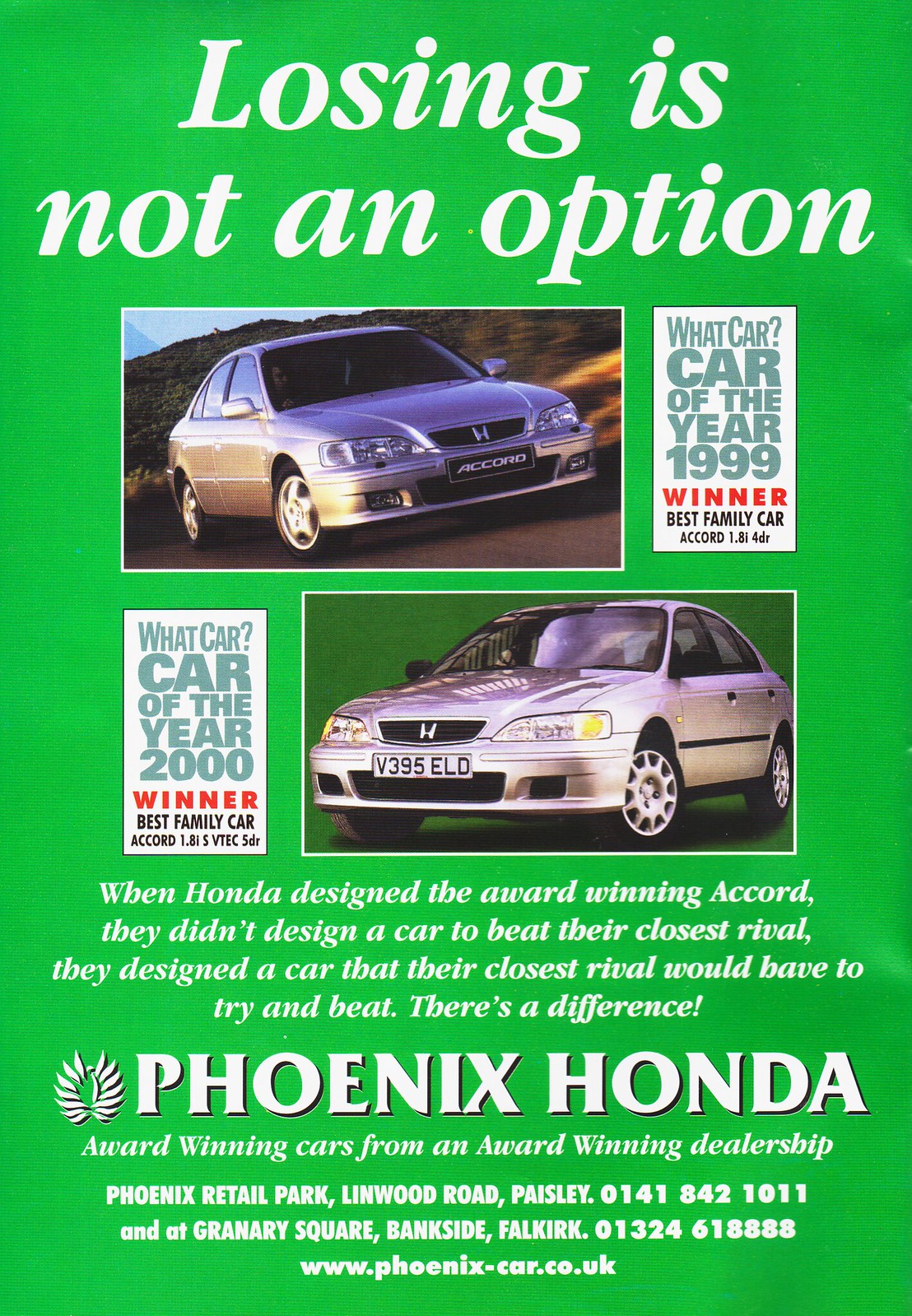The advertisement image features a clear and concise message with a striking visual design. Against a green background, the bold, white, italicized text at the top declares, "Losing is not an option." Below this phrase, the ad displays two silver Honda Accords. The first car, slightly angled to the right, has a black license plate with the word "Accord" in white letters. Positioned to the right of this vehicle, text in various colors reads: "What Car? Car of the Year 1999 Winner, Best Family Car."

Adjacent to it, another silver Honda Accord faces slightly left. This car's license plate, in contrast, features black letters on a white background that reads "V395 ELD." Directly beneath this second car, additional text proudly states, "What Car? Car of the Year 2000 Winner, Best Family Car."

Further down the poster, in smaller white text, the ad elaborates: "When Honda designed the award-winning Accord, they didn't design a car to beat the closest rival—they designed a car that their closest rival would have to try to beat. There's a difference."

The bottom of the ad prominently features the Phoenix Honda logo and the text "Phoenix Honda" in large white letters. Directly underneath, further contact information is provided, listing two dealership locations: "Phoenix Retail Park, Linwood Road, Paisley 0141 842 1011," and "Granary Square, Bankside, Falkirk 01324 618 888." The website is also mentioned, appearing as either www.phoenix-car.com, .org, or .co.uk. The tagline "Award-winning cars from award-winning dealerships" concludes the ad, emphasizing Phoenix Honda's reputation for quality and excellence.